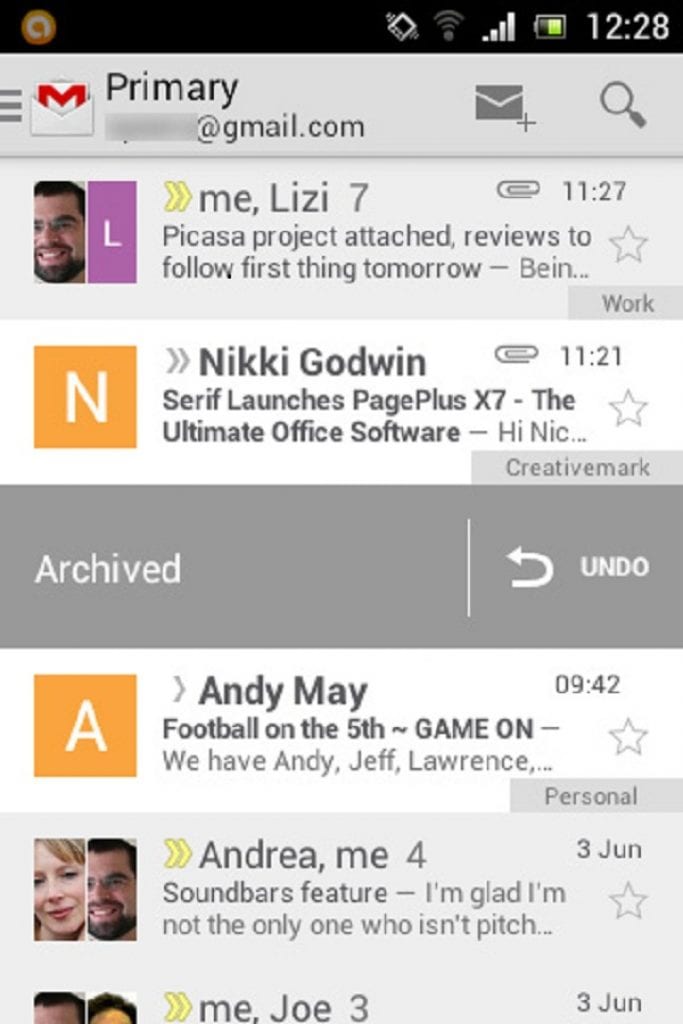The image displays a smartphone screen featuring an email application. At the very top, there's a black status bar showing standard indicators for cellular signal strength, Wi-Fi connection, and the current time. Below the status bar, the app's interface includes a primary email folder marked with a white envelope icon and a red "M," indicating a Gmail account. 

Towards the upper section of the screen, there are functional icons: an envelope with a plus sign for composing a new email, and a magnifying glass in gray for search functionality.

The main section of the screen showcases a list of emails. The first email is from "Me, Lizzie," marked with the number 7 and a paperclip icon, suggesting attachments. The timestamp reads 11:27 AM, and the subject indicates a discussion about Picasa, with pending reviews mentioned: "Picasa, projected, attached, reviews to follow, first thing tomorrow."

Following is an email from "Nikki Godwin," also with a paperclip icon, timestamped at 11:21 AM. The subject highlights a product launch: "Surfy launches PagePlus X7, the ultimate office software."

The screen also includes an archive section featuring various emails. One notable email is from "Andrew May," timestamped at 9:42 AM, labeled as personal. The email discusses plans for a football game: "Football on the 5th, game on. We have Andy, Jeff, Lawrence."

Another email, tagged with the number 4, is from "Andrea and me," dated June 3rd. The subject reads: "Soundbars feature," with the partial content stating: "I'm glad I'm not the only one who isn't pitch."

The majority of the app's interface utilizes a white or gray background with black text, with several interactive buttons scattered throughout the display.